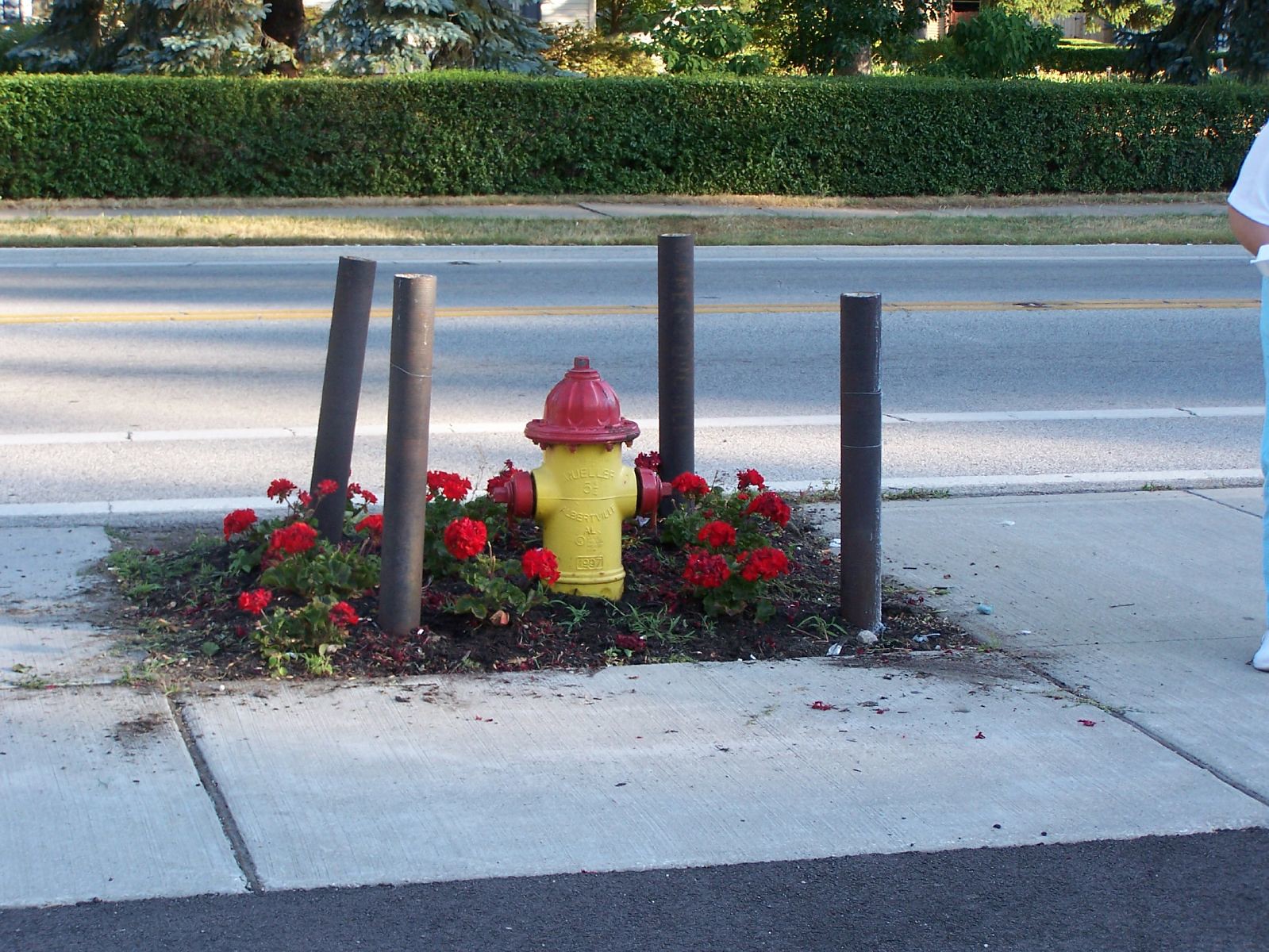In this detailed daytime photograph, likely taken in a neighborhood, the main subject is a prominent yellow fire hydrant with a red top and red side valves. This hydrant is installed in the middle of a cement sidewalk square that has been cut out and landscaped with vibrant red flowers, possibly geraniums or tulips, adding a touch of color to the scene. Surrounding the hydrant are four black metal bollards forming a protective barrier. 

The background features a well-maintained sidewalk bordered by green, pruned bushes stretching from left to right. Behind these hedges, which are about three feet tall, stand an array of trees, including pine and other leafy varieties, indicating that the season is likely spring or summer.

Further back, on the other side of the sidewalk, there is a street with blacktop pavement, marked by a double yellow center line and white bike path lines, hinting at a safe, orderly environment. A patch of green grass separates this street from the sidewalk. Also visible in the image is a person's elbow, leg, and shoe, suggesting nearby human presence. The fire hydrant has some text, possibly "Mueller," and additional markings, adding to the sense of realism in this thoughtfully captured suburban scene.